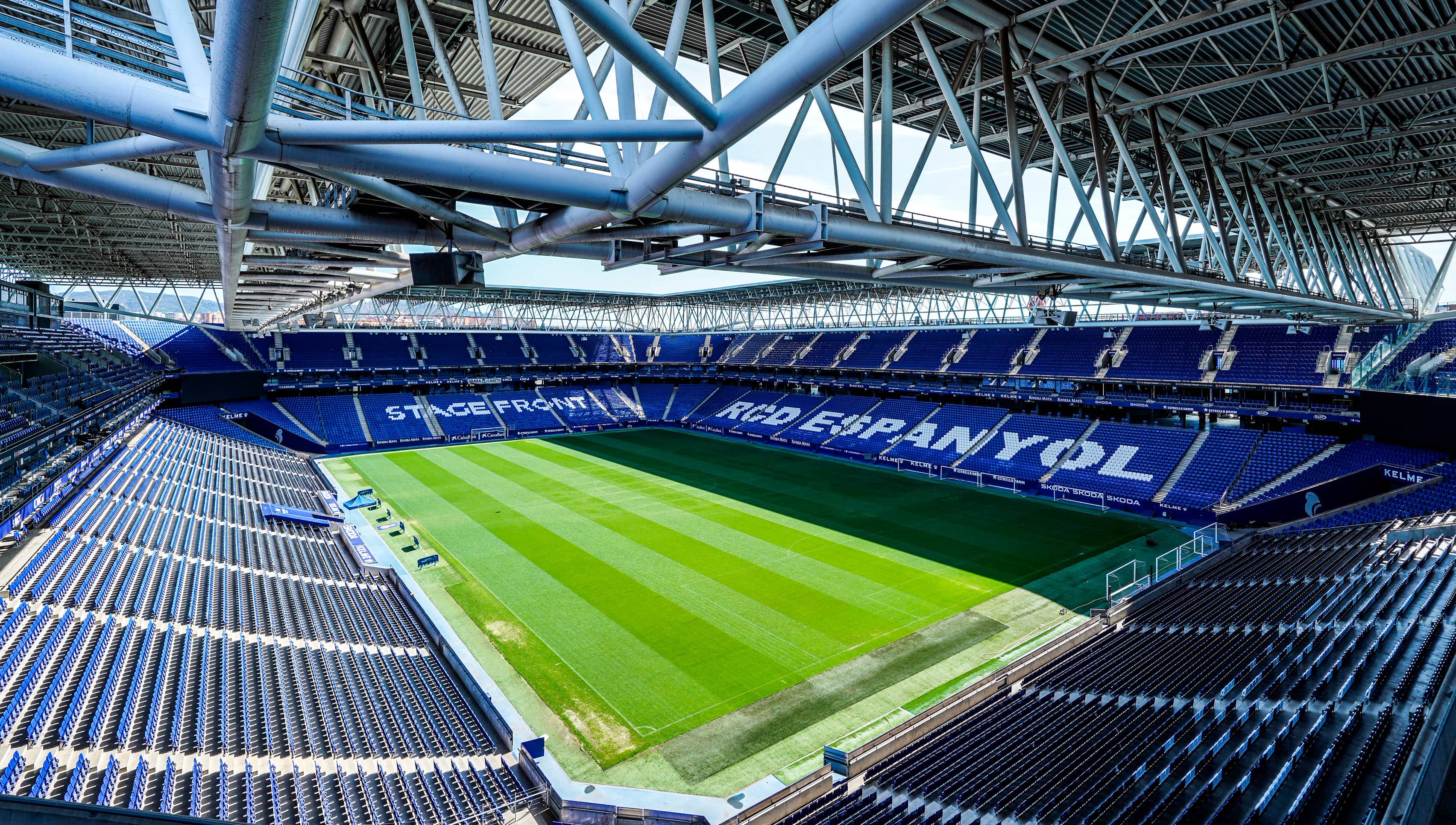An elevated wide-angle view captures the green soccer field inside a partially open-air stadium. The field boasts freshly mown grass patterned with alternating light and dark green stripes running lengthwise. The stadium seats, all in blue, encompass the lower corners and ascend to different levels, wrapping around the field. Above the seating area, the stadium features exposed industrial metal beams and a retractable roof, allowing a glimpse of the blue sky. White lettering on the seats spells out "Stage Front" and "RCD Espanol," visible even from a distance. Additionally, the left side of the field shows some equipment lined up along the sideline. The overall aesthetic of the stadium is characterized by its green pitch contrasted against a backdrop of blue seats and industrial metal architecture.